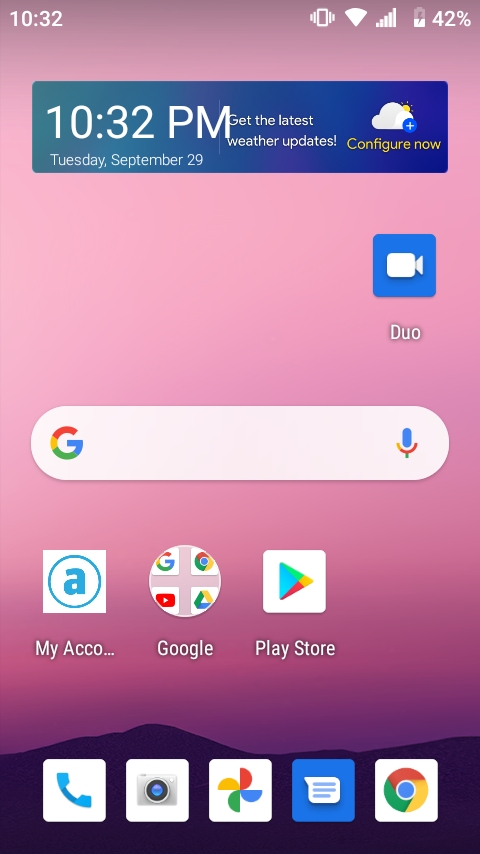Front-facing photo of a cell phone screen. The upper portion of the screen features a gradient transitioning from a pinkish-mauve hue to a deeper, more subdued color towards the bottom. The very bottom edge of the screen is nearly black, resembling the silhouette of mountains.

At the top of the screen, it's 10:32 p.m., indicated by the clock, with various icons visible, including a 42% battery icon on the right. A blue-purple-green notification rectangle displays the time 10:32 p.m., a prompt for the latest weather updates, the option to "Configure Now," and the date, "Tuesday, September 29th."

Further down, there's a dual video icon, followed by a Google search bar with a microphone icon on the right. Below the search bar, an account management icon titled "My Account" is visible. Near the bottom-center, the Google logo is displayed with additional circular icons.

On the right side, there's a Play Store icon featuring a multi-colored triangle. Lastly, at the very bottom, there are five navigation icons lined up horizontally.